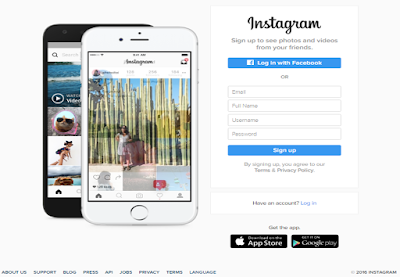In the image, on the left, there is a black smartphone displaying an ocean scene with the image of a cat overlayed on it. To the right, there is a white smartphone showing an Instagram page where a person is standing in front of a dense bamboo forest. The Instagram page appears to be an alternative iPhone view, prompting the user to sign up to see photos and videos from friends. The sign-up section includes fields for full name, username, password, and options to log in via Facebook or email. The text below indicates that by signing up, users agree to Instagram's terms and privacy policy. Additionally, there are options to get the app from the App Store or Google Play. The white background and overall style suggest that this is a promotional or instructional mock-up of an Instagram interface from around 2010. Several footer links are visible, including support, blog, press, API, jobs, privacy, terms, and language settings. The image captures the early corporatized aesthetic of Instagram, emphasizing its community and app accessibility.